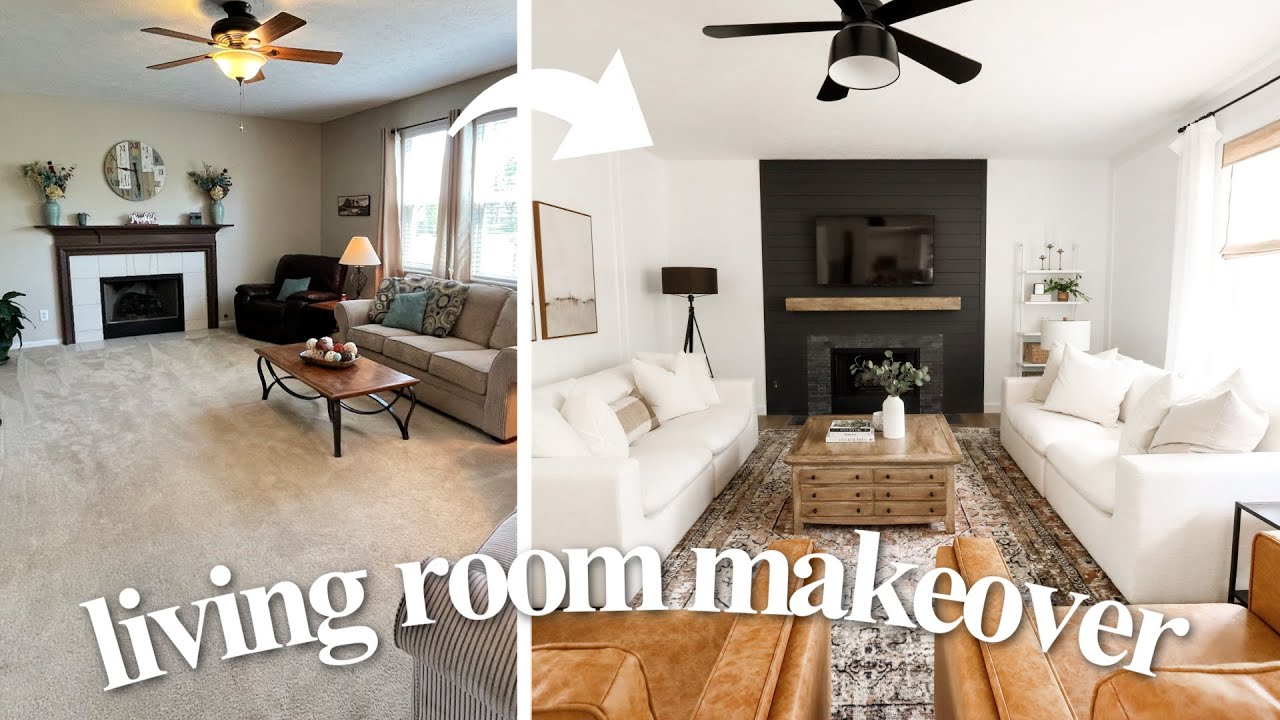This is a before-and-after photo of a living room makeover, showcased with the text "living room makeover" in lowercase white letters across the images. The "before" image on the left features a family room with a beige short carpet, light gray walls, and a ceiling fan. The décor includes a beige couch with floral pillows, a small coffee table, and a gray sofa paired with a lounge chair. There's also a dark wood mantle fireplace adorned with vases and two windows to the right.

The "after" image reveals a transformation into a fresh, modern living space. The walls are white, featuring a black painted fireplace, now more prominent in size. The room includes two modern white sofas with fluffy pillows, and two beige chairs, complemented by a stylish small square coffee table with decorations. The furniture layout introduces new elements like a different ceiling fan and a contemporary rug, enhancing the overall sleek and updated aesthetic.